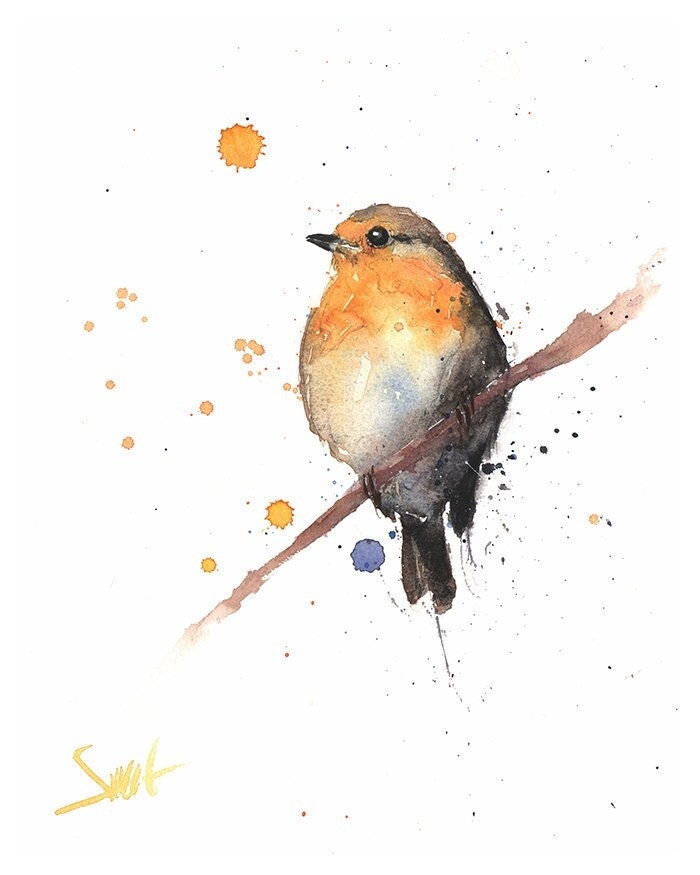This watercolor painting captures a small bird perched on a single brown branch, against a solid white background adorned with splatters of orange, yellow, blue, and black, giving it an artistic, dynamic touch. The bird, which resembles a robin or sparrow, features an orangey top with a gradient blending into a light white or nude color on its belly. It has a distinct black beak, eye, and shading along its back and tail, with two prominent black feathers extending below the branch. The bird, seen in a blurry, watercolored style, appears to be looking to the left, disengaged from the viewer. The painting is signed in yellow script at the bottom left with the word "shot," adding a personal touch from the artist.